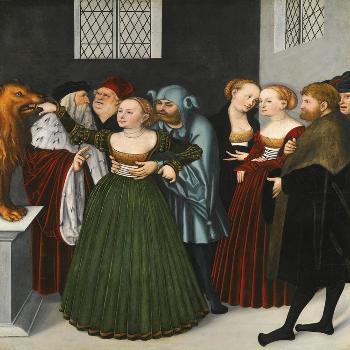The image appears to be a detailed, Victorian-era painting depicting a bustling room with several figures and interactions. Centrally, a brown dog stands on a white pedestal, gently gripping a woman's hand in its mouth. The woman, unfazed, is dressed in a long green dress with her hair neatly tied up. To her left, there are three men; two are engaged in conversation, while the third, clad in a blue cloak, is holding the woman's waist. In the right section of the painting, two women in similar dresses with white waistbands, brown tops, and maroon skirts, converse. Further to the right, two men stand together. The background features dark walls, one black and one gray, complemented by upper windows, contributing to the room's somber and historical ambiance. The scene is rich in period detail, suggesting a gathering or event evocative of the Victorian era.